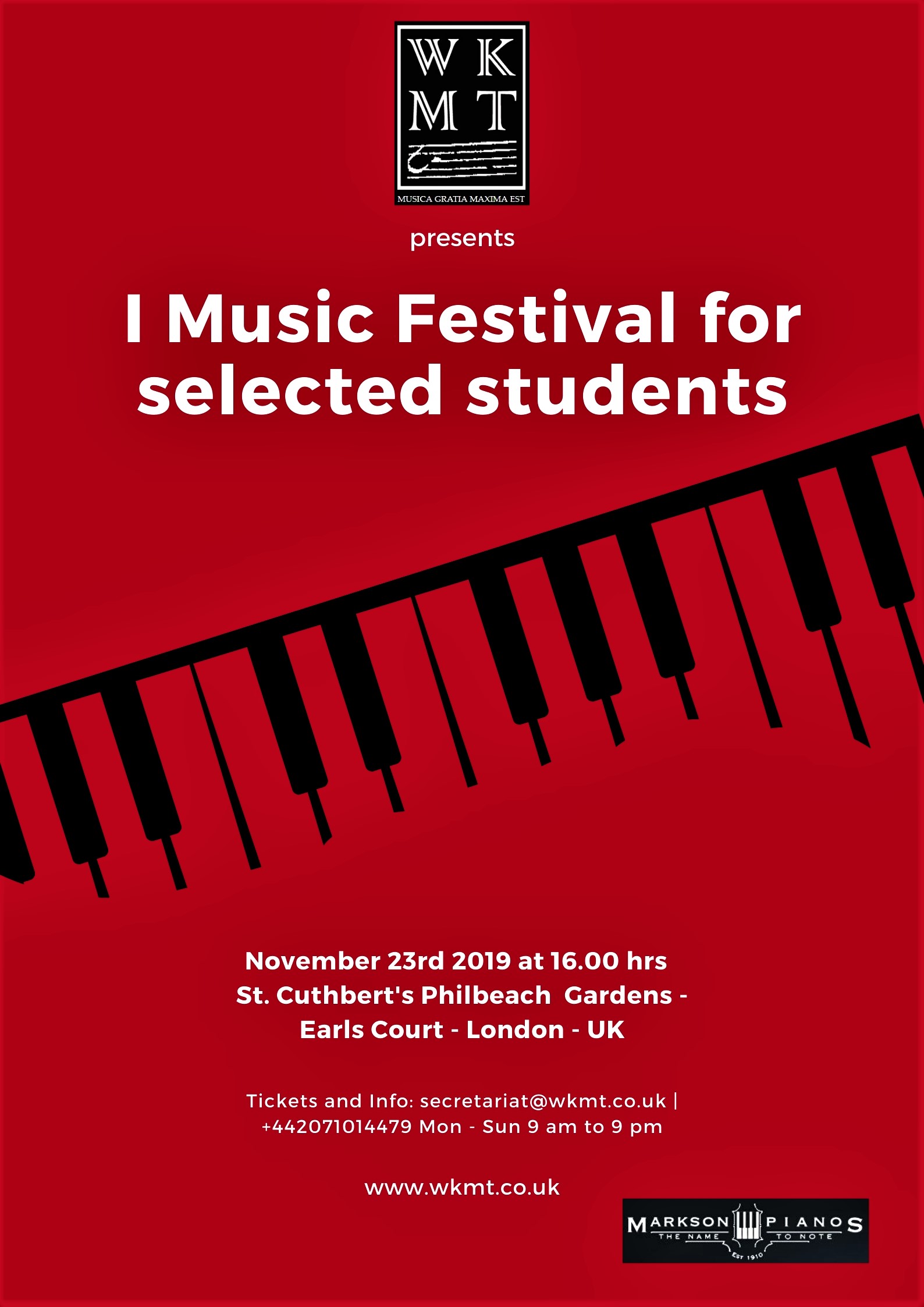The image features a prominent red rectangular background. At the top of the image, there is a black square with a white border, centrally displaying the initials "WK" in bold letters, with the subtitle "MT" just below it. Underneath, the title "Presents" is written, followed by the main event title "iMusic Festival for Selected Students" in striking white letters.

Below the text, an illustration of black piano keys is diagonally positioned, adding a musical theme to the image. Centered beneath this graphic, near the bottom, important details of the event are displayed in white text: "November 23rd, 2019 at 1600 hours, St. Cuthbert's Field Beach Gardens, Earls Court, London, UK."

Further down, smaller text provides additional information: "Tickets and Info: Secretariat at wkmt.co.uk" followed by the contact number "+44 207 101 4479, Monday through Sunday 9am to 9pm." The website "www.wkmt.co.uk" is listed at the bottom. On the right side of the image, there is a black box, balancing the composition and adding emphasis to the textual information.